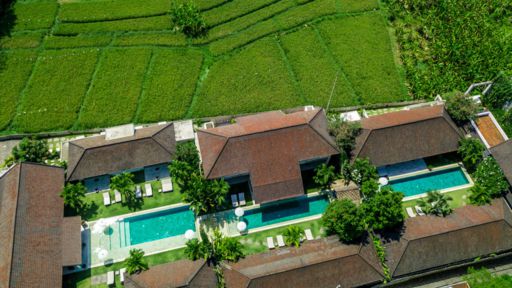This aerial photograph, taken from a helicopter or plane, presents a detailed bird's-eye view of a residential complex consisting of eight houses arranged in a rectangular formation. The houses feature brownish-reddish roofs with a distinctive triangular shape, curving upward towards a central ridge. Nestled in the middle of these homes is a large, rectangular swimming pool enclosed by white walls, filled with vibrant bluish-green water. Adjacent to the pool are several white beach chairs, adding a touch of leisure to the scene. The top half of the image showcases a wide expanse of neatly mowed lawns with pathways traversing through it, leading to a tree situated at the very top of the photograph. The right side of the image is bordered by a dense cluster of trees and bushes, juxtaposing the structured greenery around the houses.